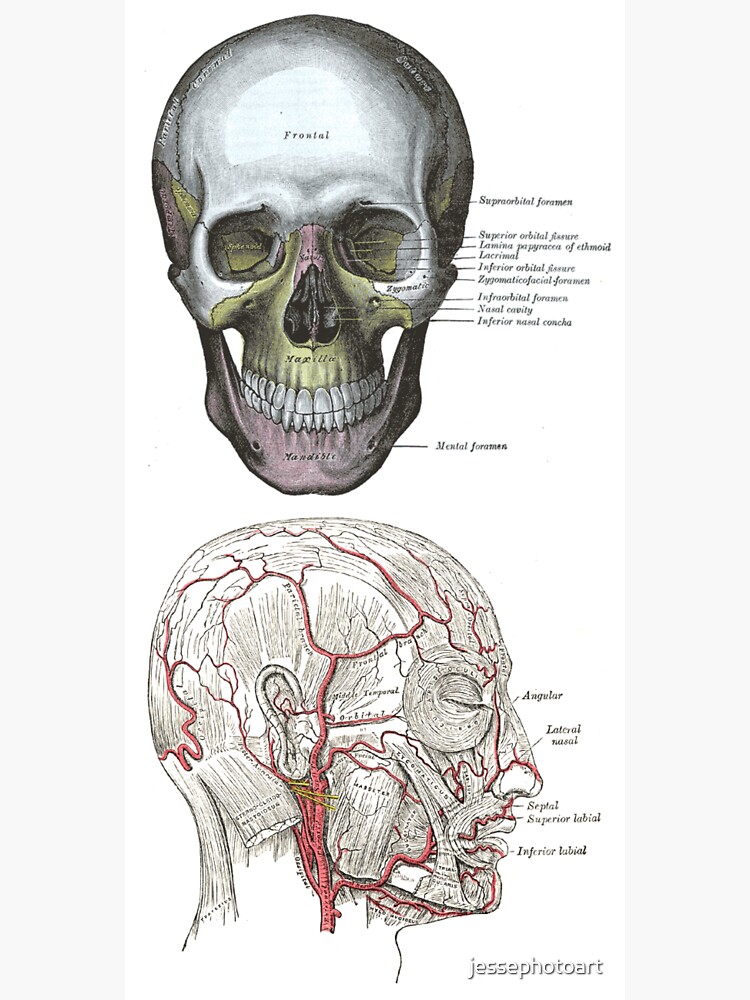The image is a detailed anatomical illustration from an actual anatomy book, credited to Jesse Photo Art. It features two separate depictions of the human head. The first image, positioned at the top, is a forward-facing view of a human skull. The skull is color-coded in shades of gray, dark yellow, and light red, with lines pointing to and labeling each bone structure, such as the teeth and eye sockets.

The second image, situated below, is a side profile of a human head. This profile appears translucent, revealing the complex network of arteries and veins beneath the skin. The veins are depicted in red, accompanied by labels for specific vessels, including the angular lateral nasal septal, superior labial, and inferior labial arteries. Additional labels identify facial features such as the nose, lips, and closed eye, and the positioning of the ear.

Both images are intricately sectioned and categorized, providing a comprehensive view of the skeletal and vascular systems of the head. The bottom right corner of the illustration bears the name 'Jesse Photo Art,' attributing the creation and online sharing of this detailed educational resource.